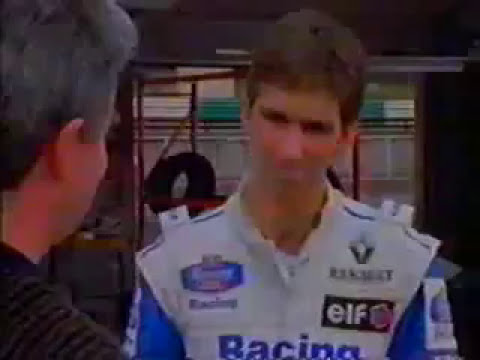In a blurry, low-resolution screenshot, a young man stands on the right, facing an older man on the left. The young man, who has short brown hair and white skin, is clad in a white racing vest adorned with various brand logos, blue sleeves, and a blue shirt underneath, decorated with indiscernible white symbols. Prominently, the chest area reads "Racing" in blue text. He's smiling slightly, without showing his teeth. The older man, only partially visible, has gray hair that's about three to four inches tall and noticeably rosy cheeks and ear. He wears a black shirt. Surrounding them is a backdrop featuring a black tire, a dark opening like a garage door, and a wall covered with papers and posters.